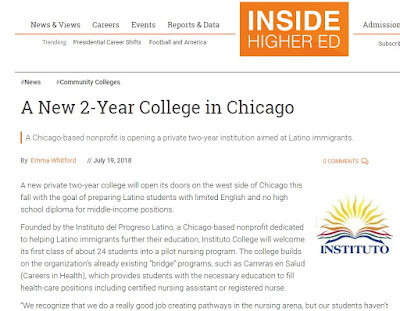This is an image of a news article from Inside Higher Ed, titled "A New Two-Year College in Chicago," published on July 19, 2018, and authored by Emma Whiteford. The article discusses the opening of a private two-year institution in Chicago, specifically designed to support Latino immigrants. The initiative is spearheaded by the Instituto del Progreso Latino, a Chicago-based nonprofit organization dedicated to advancing the educational prospects of Latino immigrants. The college has launched with a pilot nursing program accepting 24 students this fall. It aims to provide opportunities for Latino students who have limited English proficiency and no high school diploma to secure mid-income jobs, emphasizing the importance of accessible educational pathways for this community.